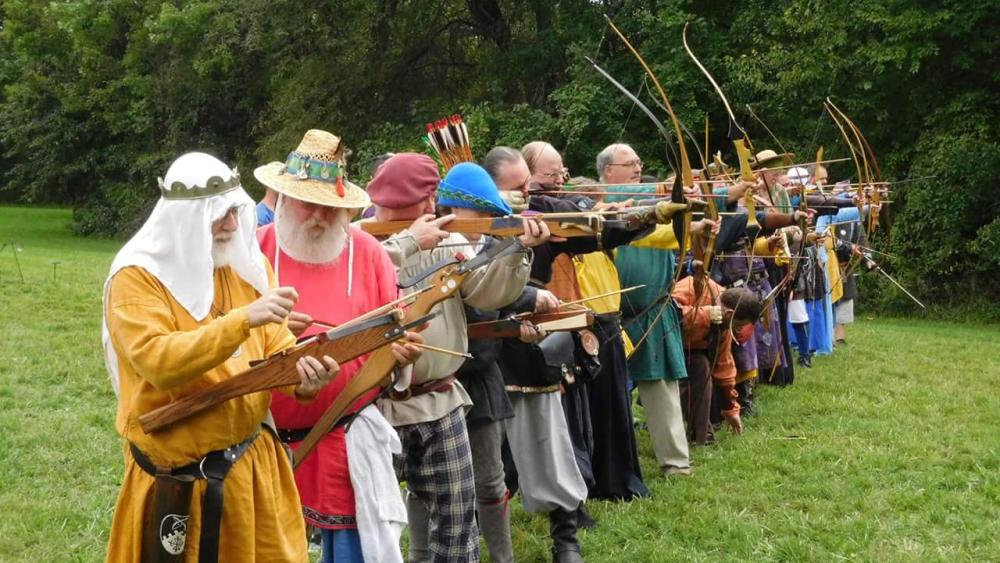The photograph captures a line of approximately 15 older men, likely in their 60s and up, standing on a grassy lawn with a dense forest backdrop, possibly at a Renaissance fair or festival. The men are dressed in an eclectic mix of costumes from various historical periods. Starting from the left, a man dressed as a sheik wears a yellow tunic with a white head covering and a crown, with a black belt and a white beard. To his right, another bearded man in a pink or salmon-colored tunic with a straw hat and crossbow stands out. As the line progresses, the first half of the men, about six of them, are equipped with crossbows and dressed somewhat like Friar Tuck with medieval garments. The latter half transitions to men holding traditional tall bows, poised as if ready to shoot, signifying a shift from crossbowmen to archers. Their costumes range from mustard yellow to burgundy and include various hats like straw, berets, and velvet caps. Some men are balding or wear glasses, and their attire includes long pants or tall socks with knee-length trousers. The photograph is angled slightly, giving it a dynamic look, and the collective image suggests a ceremonial or organized display, possibly for a historical reenactment or defense line.